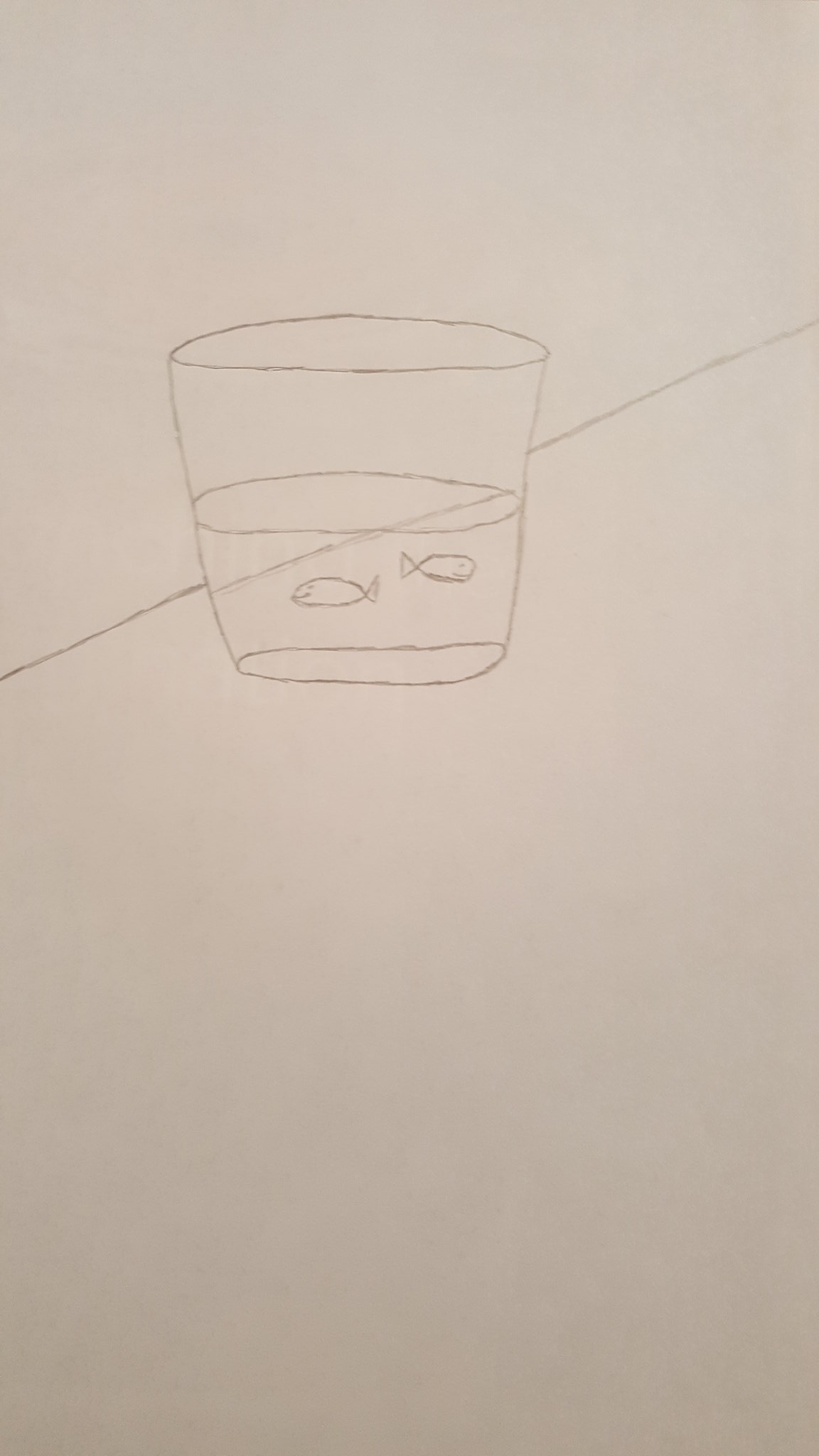In the image, a white cup is depicted with two intricately drawn goldfish swimming inside it. The cup contains a liquid, with a chili straw sticking out, adding a vibrant touch to the scene. A black line bisects the top left corner of the frame, providing an abstract element to the otherwise minimalist background. The overall setting is against a pristine white backdrop, accentuating the simple, yet compelling, black line drawings within and around the cup.